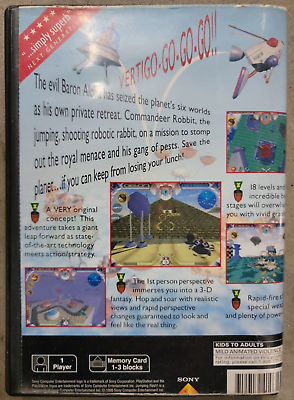The image is a detailed photograph of the back cover of a PlayStation video game box. The layout is vertically oriented, with prominent elements including a red diagonal banner in the top left corner featuring five stars and the phrase "simply superb" in white text, followed by "next generation" in black. At the top center, red text reads "Vertigo, go, go, go," set against a blue sky background with flying robots and UFOs. 

The main description outlines the evil Baron seizing the planet and its six worlds, retreating to his private domain. The player controls Commander Rabbit, a jumping, shooting robotic rabbit on a mission to eliminate the royal menace and his gang of pests. The text whimsically adds, "Save the planet if you can keep from losing your lunch."

At the bottom, practical game information is displayed: "one player," "memory card 1-3 blocks," and the Sony PlayStation logo. Additionally, there is a rating of mild animated violence suitable for kids to adults. The back cover is adorned with four small screenshots showcasing game environments such as a yellow pyramid and green grass, each accompanied by descriptive icons and texts.